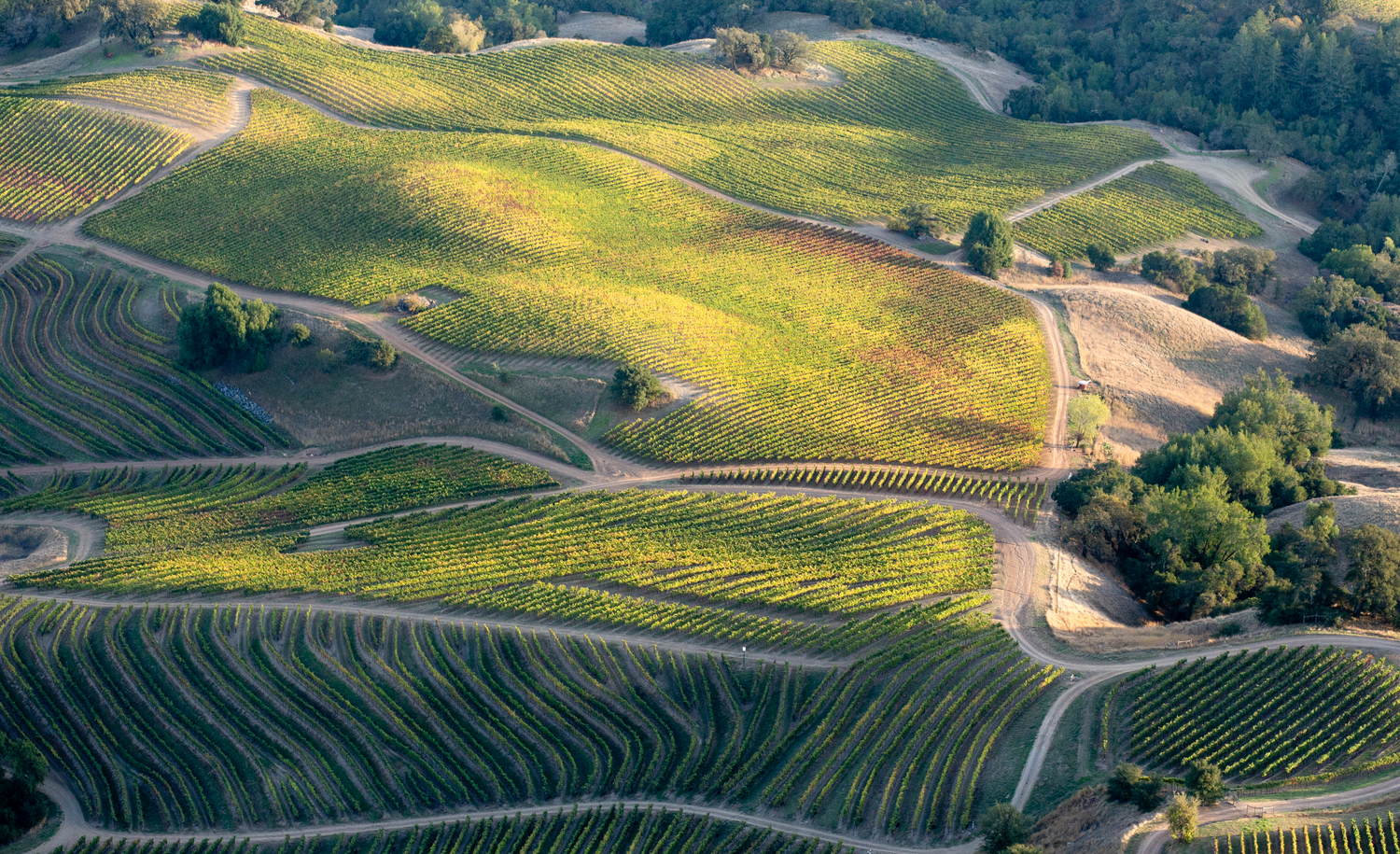This aerial view photograph depicts a sprawling landscape divided into irregular, organic-shaped sections, bordered by dirt roads. The large field, likely a farm or vineyard, features meticulously organized rows of crops, possibly grapes, interspersed with paths for access. Patches of green grass and numerous trees populate the right side and backdrop of the image. The sun illuminates the scene, highlighting the contrast between the sections of planted rows, walking lanes, and expanses of grassy areas. There are no visible buildings, emphasizing the natural and agricultural expanse of this vibrant, sunlit plantation.